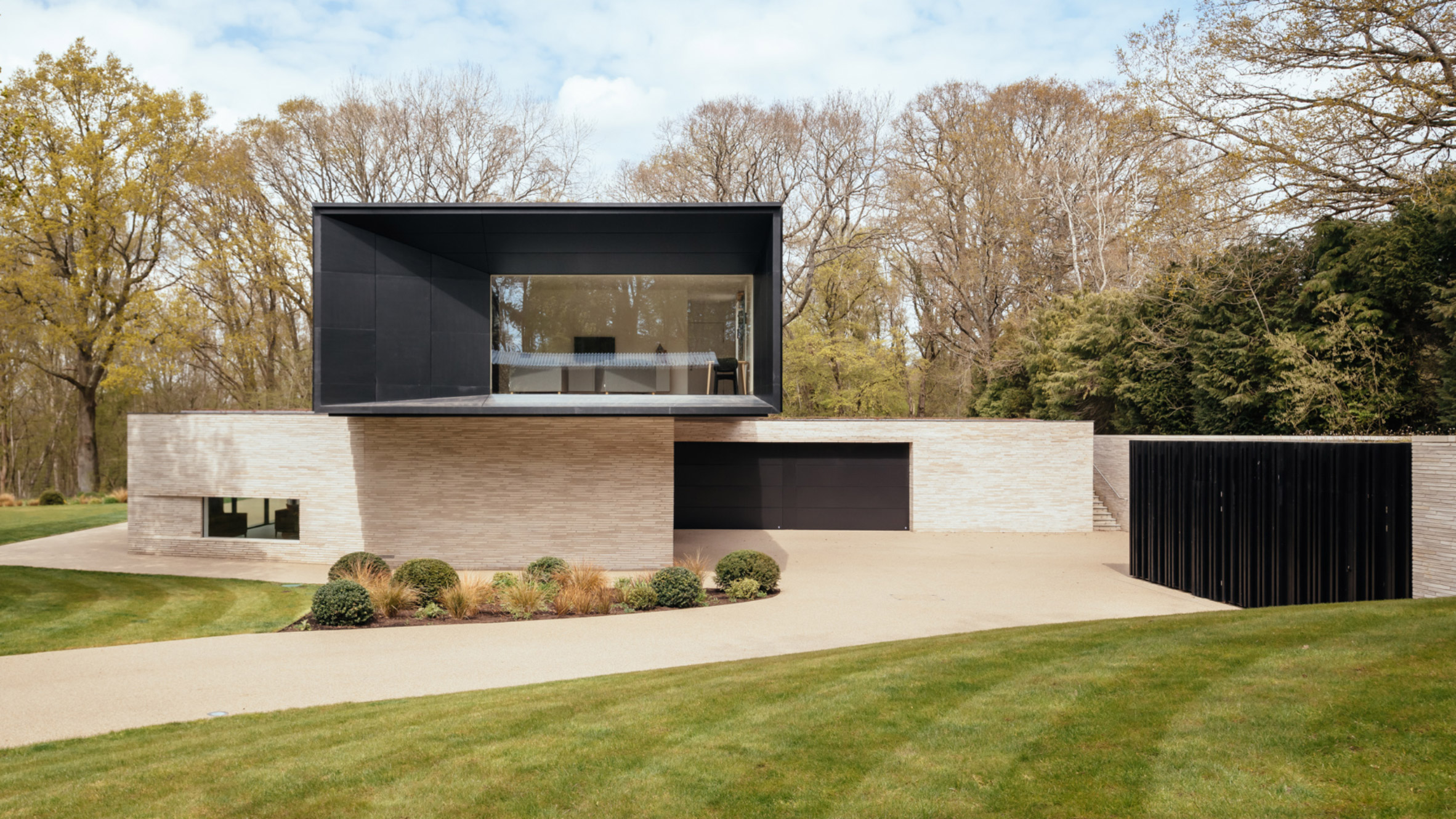This photograph showcases a very modern, simplistic, and architecturally unique home, characterized by a series of interconnected rectangular structures. The house features a distinctive two-story design where an upper black rectangular section with large windows sits atop a wider, shorter, and lighter brick lower section. There is visible furniture inside the upper section, including a couple of gray chairs and what might be a TV, though it's difficult to be certain due to glare. On the right side of this large window, there's a piece of black furniture with gold sides and possibly a doorway behind it.

The lower section of the house features a small, darkened window and has a partial shadow indicating the upper section projects outward slightly. Adjacent to this, there’s an expansive black rectangular element, possibly a garage door, with a barely visible seam, and a large metal-like black rectangular box set on a cement walkway. The grass surrounding the house is freshly mowed, creating an alternating pattern of lighter and darker green stripes. The driveway curves from the bottom left of the image past green bushes and leads up to this distinctive building.

In the background, there are sparse and yellowed deciduous trees, suggesting an autumn setting, and several evergreen firs. The sky is partly cloudy with patches of blue visible. A stairway on the right provides access to the second level, further indicating the house's elevated design. The combination of modern materials and minimalistic design elements against the backdrop of a lightly clouded sky highlights the home's contemporary aesthetic.